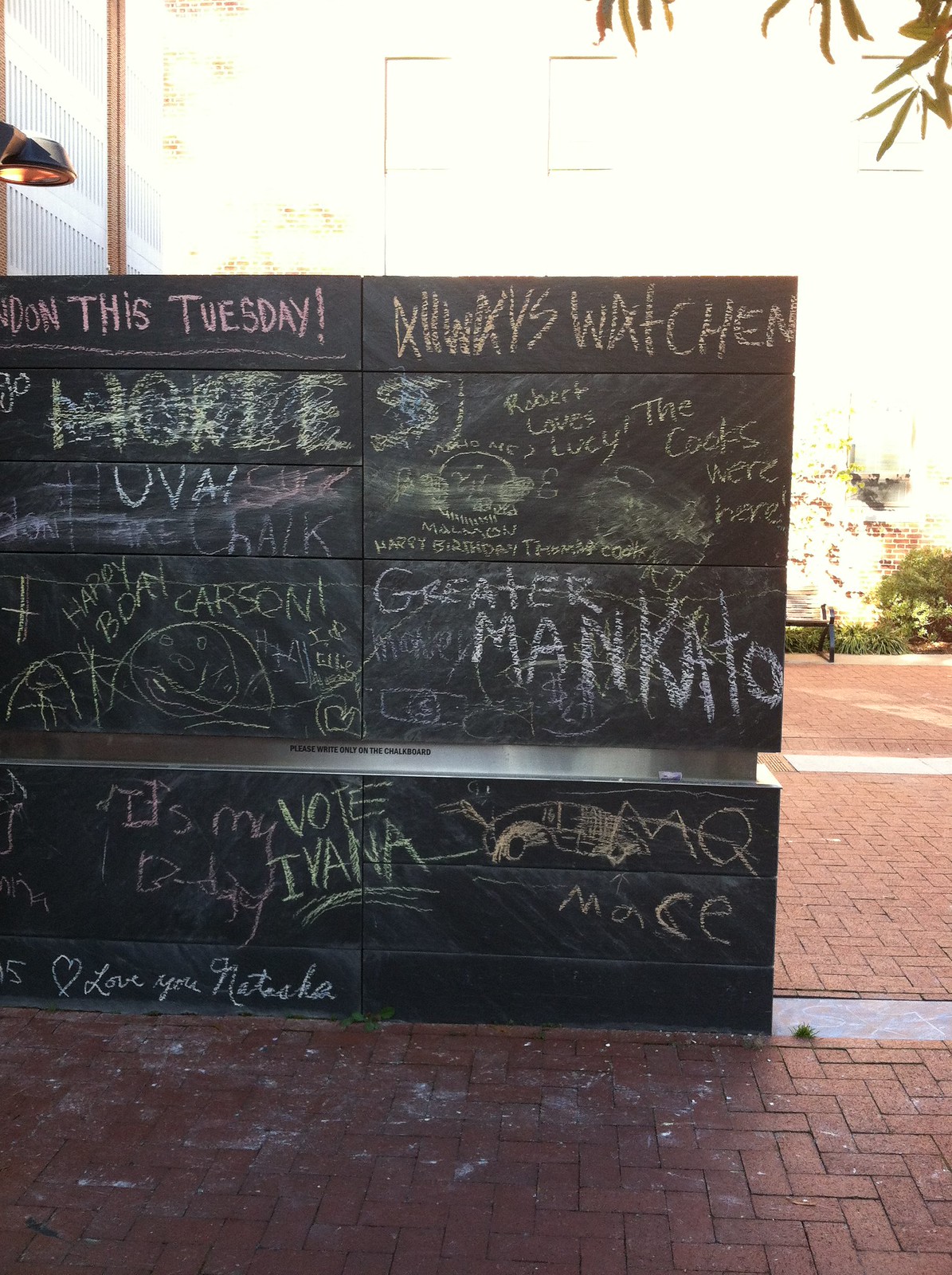An outdoor scene showcases a sunlit area with white walls and tree leaves hanging down, partially obscuring the top right corner of the image. The ground is composed of red bricks forming a walkway that extends from the foreground all the way back to a large white building. Central to the photograph is a black chalkboard covered in a mix of colorful chalk writings and doodles, including legible phrases such as "love you Natasha" in white chalk, "this Tuesday!" and "always watchen" at the top, as well as "happy B-Day Carson." The board appears messy, with many scribbles, erased sections, and chalk dust scattered at its base, giving it a slightly vandalized yet lively look. The background, though bright and a bit overexposed, hints at additional brick elements on the building's wall.